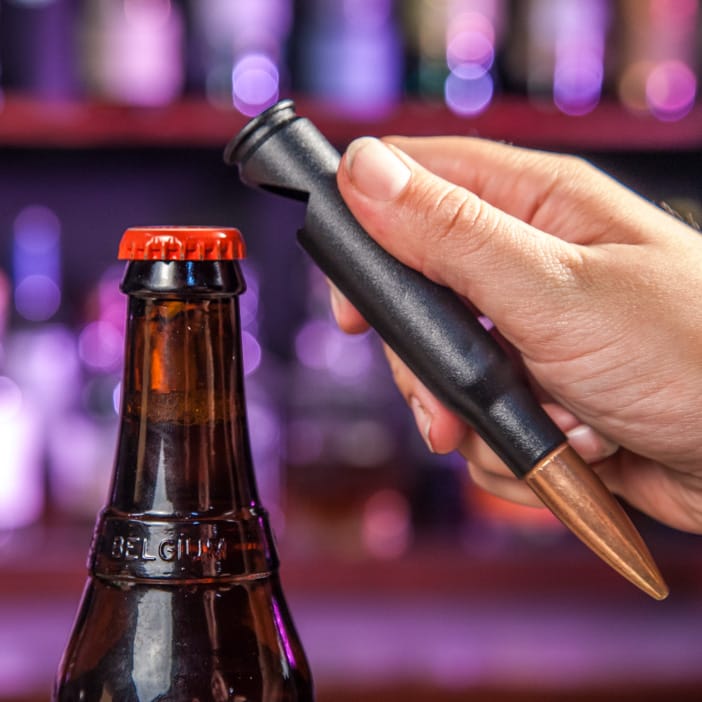The photograph captures a moment at a bar where a male hand, holding a bottle opener shaped like a large bullet, is about to open a dark brown beer bottle with a red cap. The opener features a black body with a copper tip and is approximately six to seven inches long. The label on the bottle hints that it might be Belgian beer. Behind the bottle and the hand, the blurred background reveals shelves lined with the silhouettes of other bottles, further suggesting the setting is a bar.